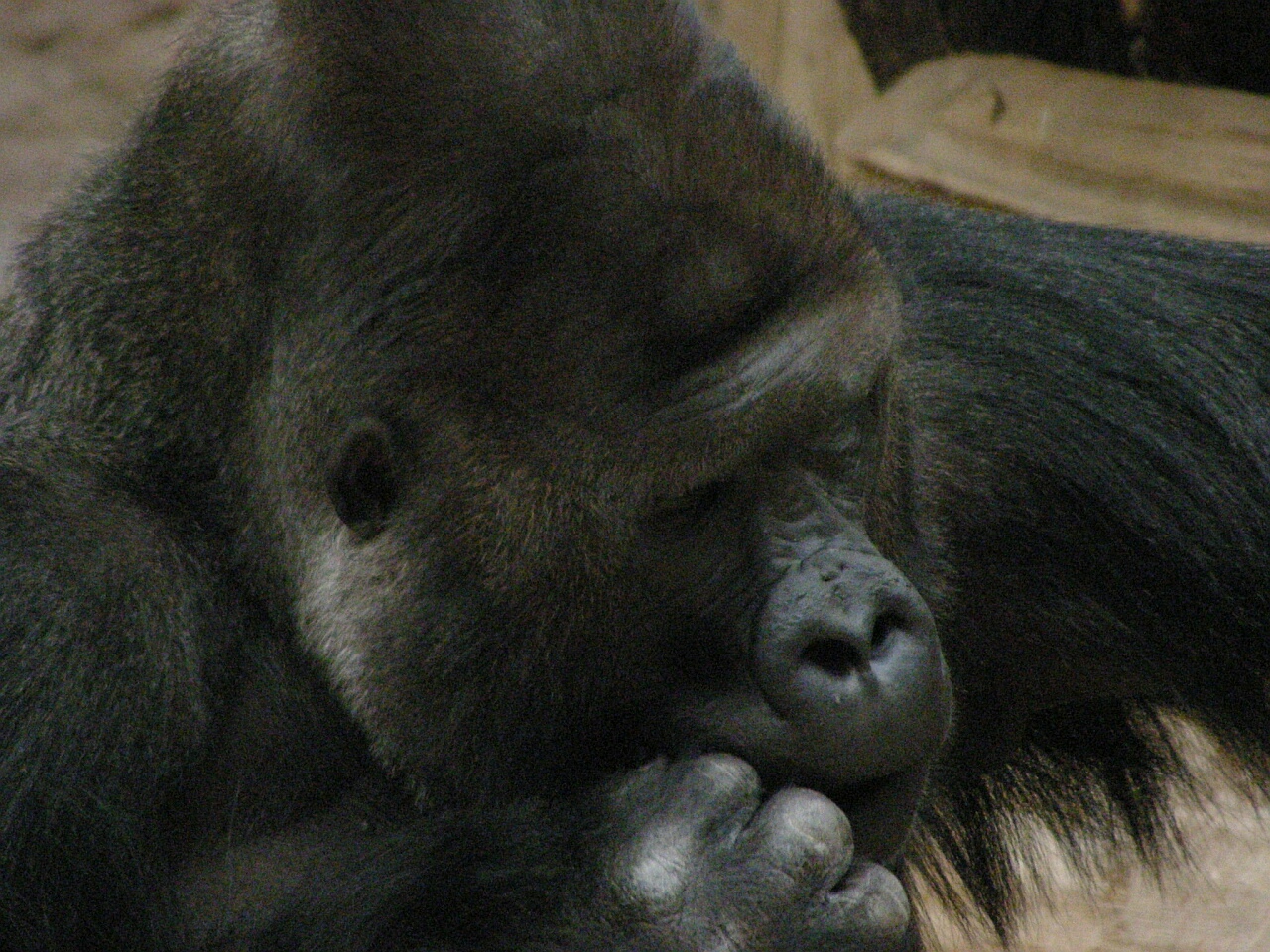This image captures a detailed close-up of a gorilla, prominently displaying the right side of its face. The gorilla is sitting, somewhat introspective, with its right hand curled into a fist near its nose. Its dark black fur appears plush and has variations in length; it is longer on the arms and shorter, slightly lighter on the head and upper shoulder, extending to a visible part of the chest. His ears are small, with the right ear clearly visible, and his facial expression is neutral, with a partially open mouth as if caught in mid-thought. The background features tan-colored rocks, and a black area behind them adds depth to the composition. It is difficult to determine whether the setting is a zoo or the wild but suggests a contemplative, possibly somber mood.